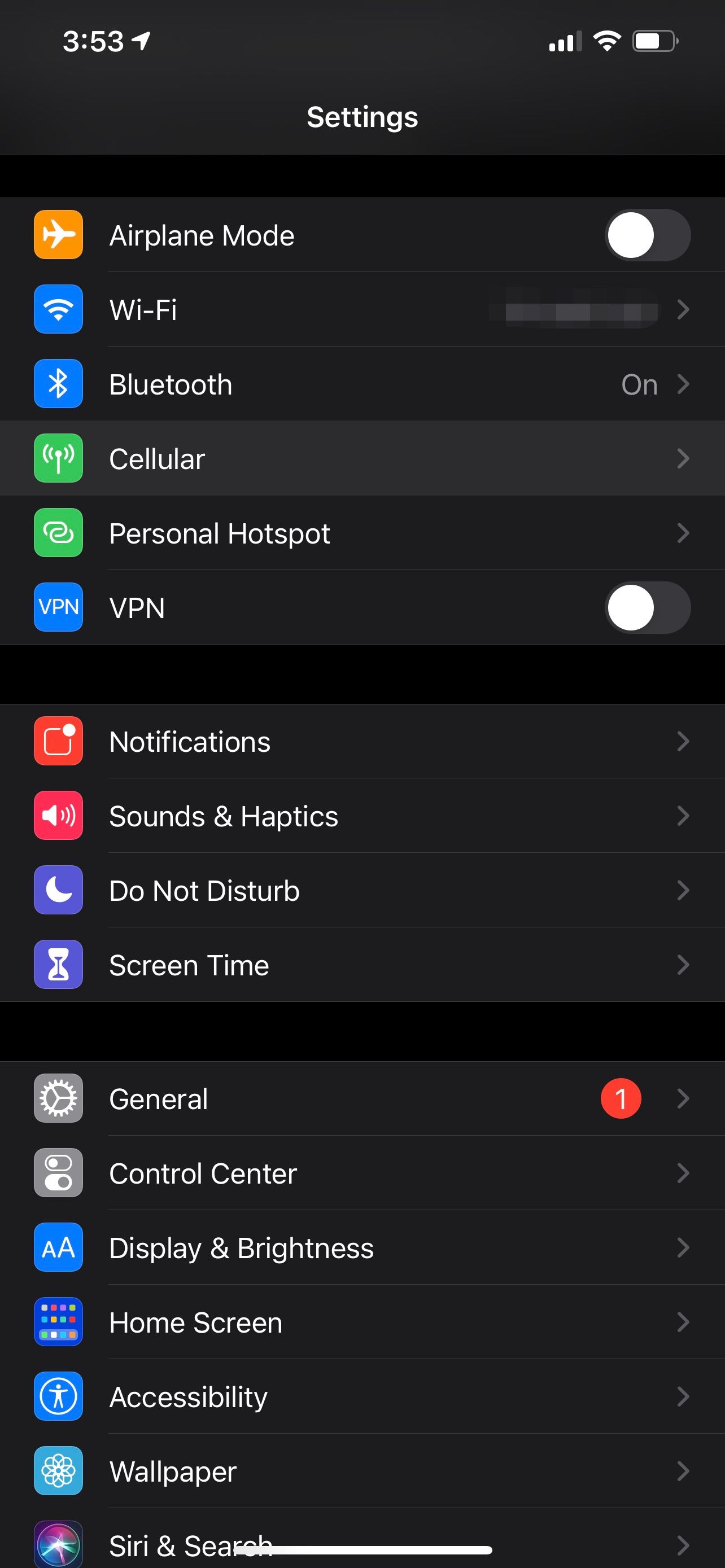The image depicts a screenshot from a smartphone displaying its settings menu. The background is predominantly black, highlighting the various settings options. At the top section of the screen, you can see the following options in order: Airplane Mode, Wi-Fi, Bluetooth, Cellular, Personal Hotspot, and VPN. Notably, Airplane Mode and VPN have toggle switches next to them, both in the off position with the white circles aligned to the left. The Wi-Fi option has its details blurred out.

A black divider separates this section from the next, which lists Notifications, Sounds & Haptics, Do Not Disturb, and Screen Time. Below another similar black divider, additional options are visible: General, Control Center, Display & Brightness, Home Screen, Accessibility, and Wallpaper. 

Towards the very bottom of the screen, partially obscured by a white line, the text "Siri & Search" is faintly visible. The right side of the screen prominently displays the aforementioned toggle switches, emphasizing the inactive status of Airplane Mode and VPN.